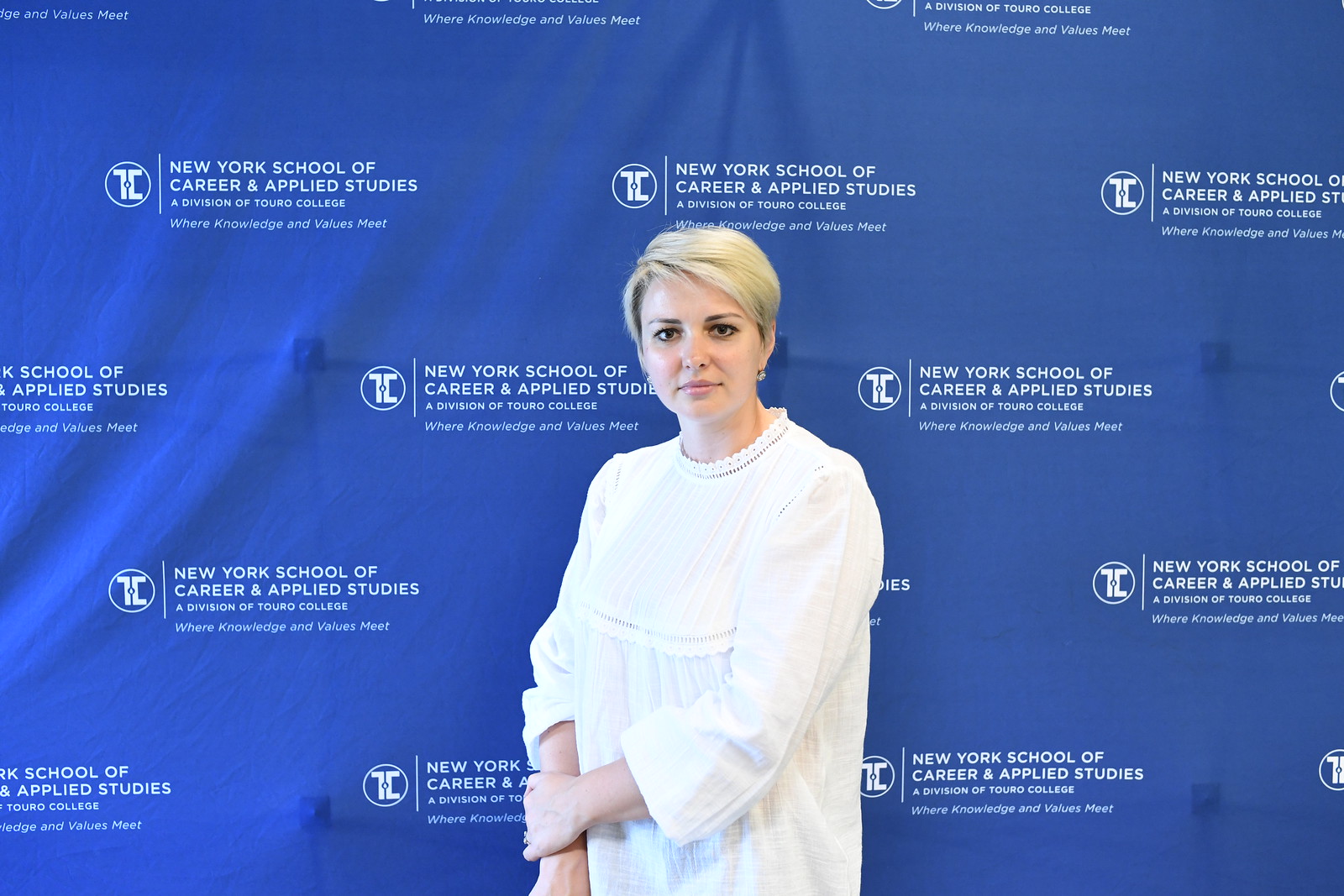A young lady stands before a blue fabric backdrop adorned with strategically-placed, symmetrical advertisements for the New York School of Career and Applied Studies, a division of Touro College, where knowledge and values meet. Her short blonde hair, parted on the left, sweeps to the right and just grazes her forehead. She has brown eyes, black eyebrows, and pink-colored lips forming a subtle, almost neutral expression. Dressed in a loose-fitting white dress with lace detail around the neckline and oversized sleeves resembling a nightgown, she also wears a pearl choker necklace. One hand is held across her chest, clasping her wrist, while the other hand hangs down by her side. The backdrop features a repeated emblem with a combined "T" and "C" inside a circle, reinforcing the institutional branding. Her poised stance and attire suggest she might be at a graduation event or a formal reception, perhaps as a VIP.